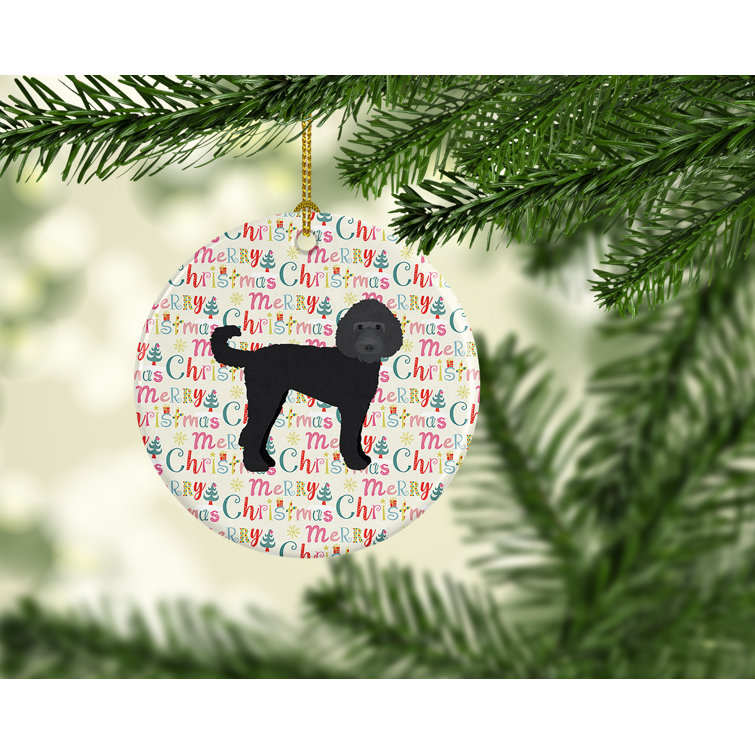In this close-up color photograph, a Christmas tree ornament takes center stage, suspended delicately by a gold string from a branch of a vibrant, artificial pine tree. The bright green plastic pine needles frame the ornament while the background fades into a soft blur of additional branches. The ornament itself is a round white disc, adorned with the repeating phrase "Merry Christmas" in an array of festive colors, including pink, blue, green, yellow, and red. Scattered among the cheerful text are small illustrations of Christmas trees. Dominating the center of the ornament is a detailed image of a black poodle. The poodle, standing upright with its tail curled to the left, gazes directly forward with its jet-black eyes and nose, its deep gray head contrasting slightly against its dark black body, bringing a touch of canine charm to the holiday décor.